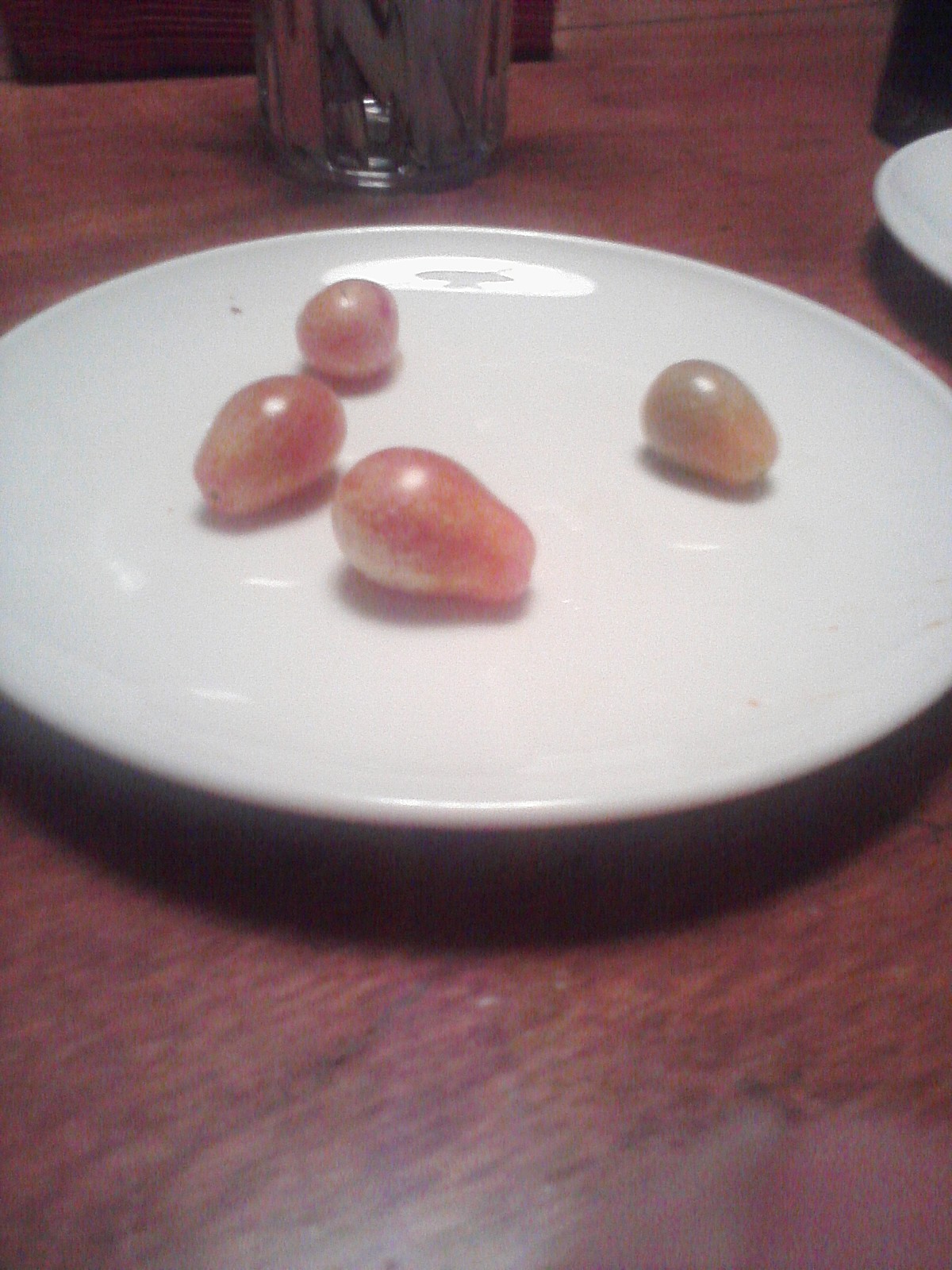The photograph features a white plate positioned centrally on a dark brown timber wood table. On the plate lies a cluster of four oval-shaped objects, resembling grapes or small tomatoes; they are red and have no stems. To the top right corner of the image, a small part of another white plate is visible. Additionally, a transparent bowl with a silver bottom is stationed at the top of the image. The main plate and the fruit on it reflect light, possibly from an overhead lamp. The entire setup creates an impression with the background's rich cherry wood tones complementing the simplicity of the plate and its contents.